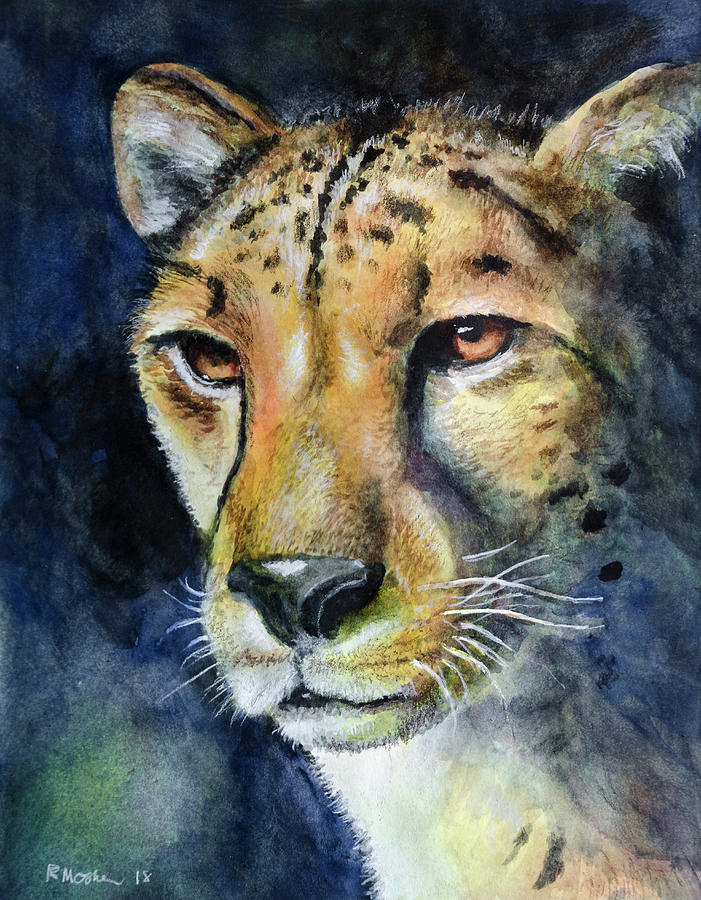This is a detailed painting of a big cat, which, based on certain characteristics, appears to be a female lion. The lion is portrayed in a portrait view, facing slightly to the left of the painter's perspective with a gaze that suggests she is looking into the distance. Her eyes—narrowed and pinkish or golden—convey intensity without aggression. Her black nose is shiny, and her snout features white whiskers. The face is mainly a yellowish-brown color with some peach and green tones, and she has black spots on her forehead. The lion's ears are perked up, indicating alertness. Her long neck extends to the right in the lower part of the painting. The background is a blend of dark blue, muted gray, white, and light green, which contrasts with the vivid, nearly three-dimensional depiction of the lion’s head. The artist's signature, "R. Mosha" or possibly "R. Moshia," is found in the lower left-hand corner alongside the number 18.